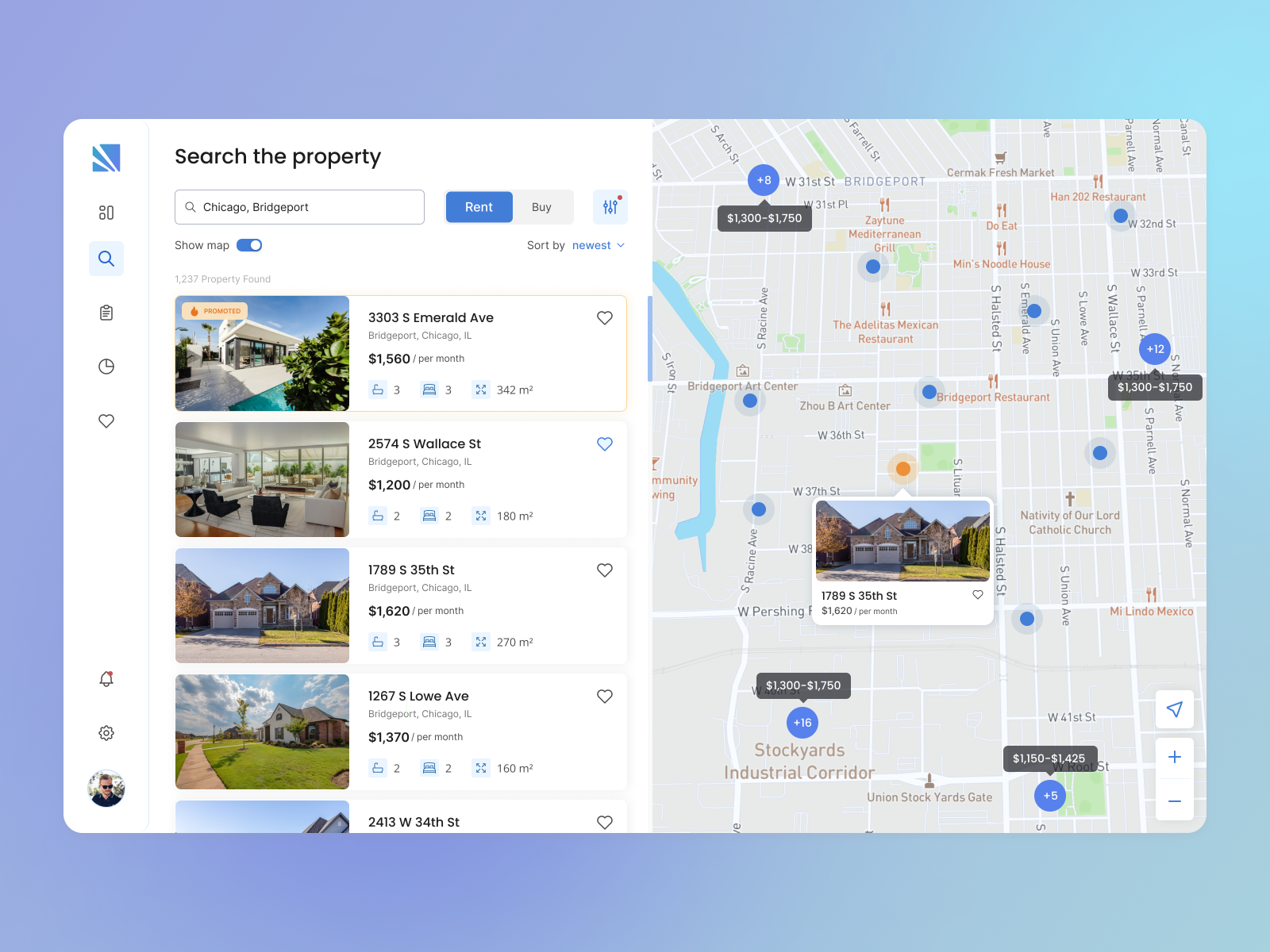A mobile application interface displaying real estate listings. The background features a gradient transitioning from purple to light teal, with a darker teal shade at the bottom. On the left side, there is a small vertical navigation menu, followed by a slightly larger search panel labeled "Search Property." The top section contains input fields for search criteria. 

To the right, there's an interactive map showing various street layouts. Several circles mark locations, most of which are blue with gray, transparent borders. The focal point, however, is an orange circle with a light orange, transparent border. Inside this circle, the address "1789 S 35th Street" is displayed. 

Below the address, the property price "$1,620 per month" is shown next to a small heart icon, which remains white like the card's background. A thumbnail image of the corresponding home is placed above this information.